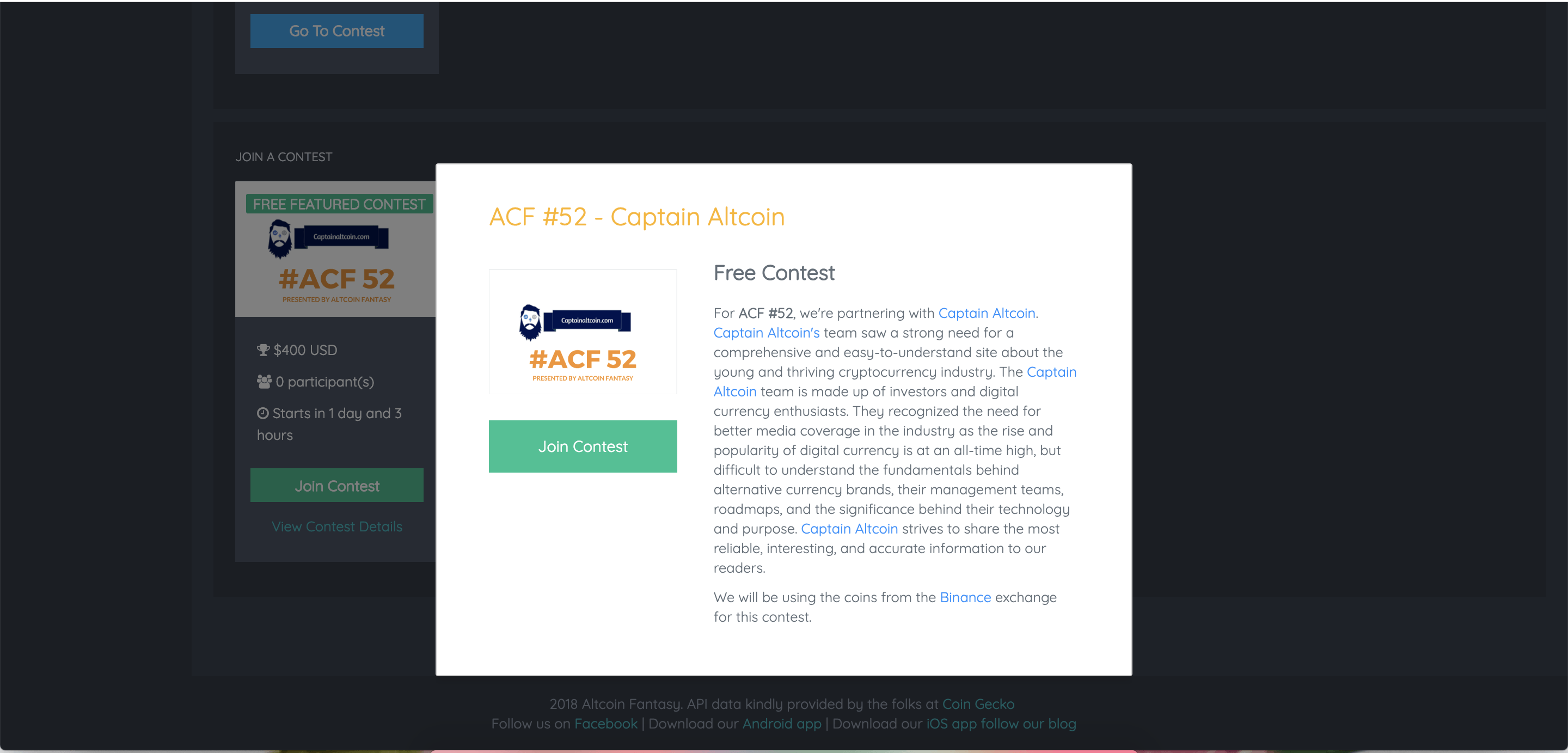The image features a central pop-up at the top left of the frame that reads "ACF-52-CaptainAltCoin" with a small box beneath it that displays "#ACF52" alongside a dark blue logo of a bearded face. Below this, there is another green box with the text "Join Contest" in white. On the right side of the pop-up, a section begins with "Free Contest" followed by a paragraph explaining that for ACF-52, they are partnering with CaptainAltCoin. CaptainAltCoin's team identified a need for a comprehensive and easy-to-understand site focused on the burgeoning cryptocurrency industry. In the background of the image, the right side is mostly empty, but on the top left, there is a blue rectangular box containing the words "GoToContest" in white text, with "Join a Contest" written below it.